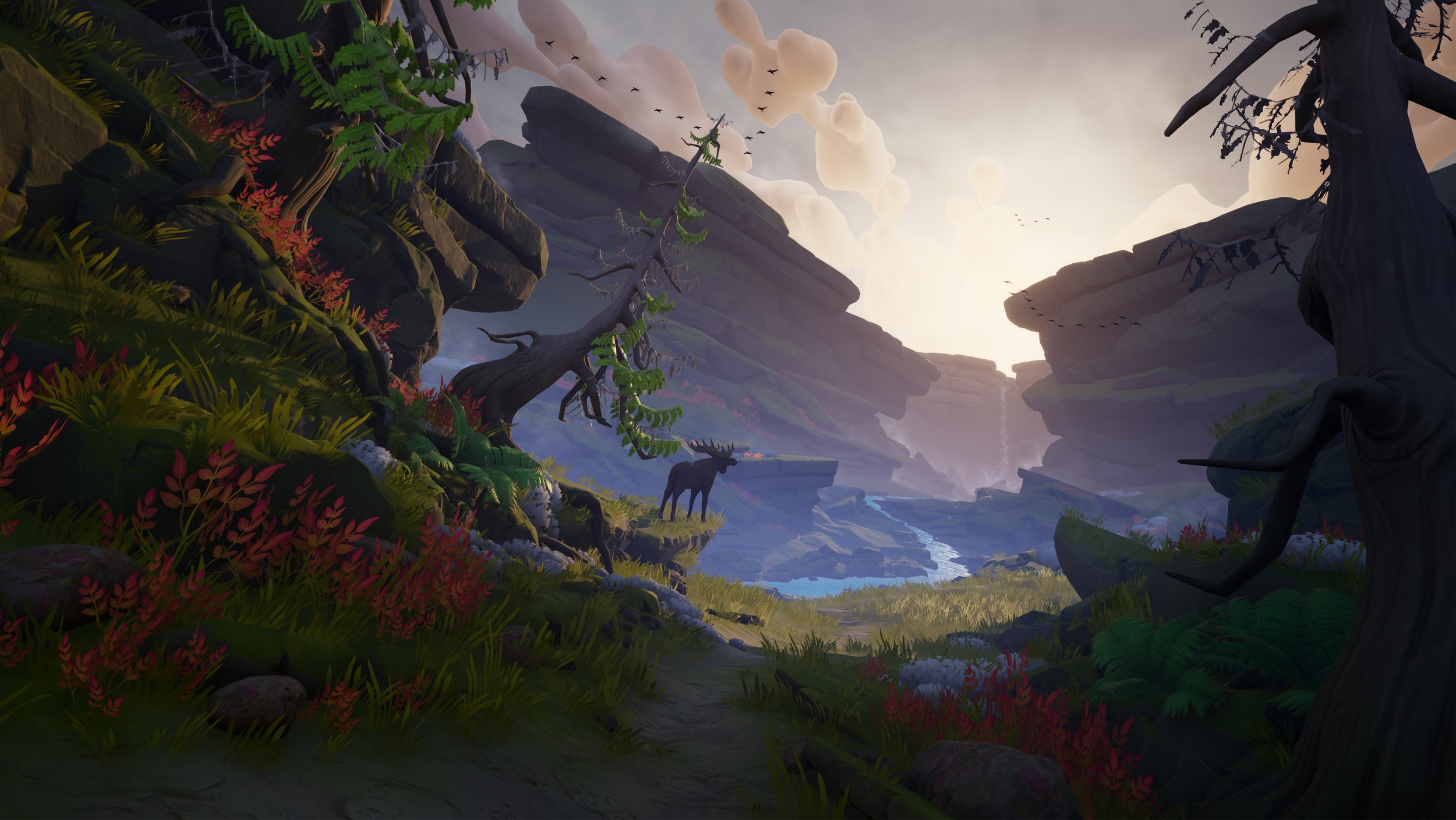In this stylized illustration, a majestic elk stands prominently at the center of the image on a promontory. The elk, viewed from behind, overlooks a scenic valley where a river meanders through curvy, animated mountain formations. To its right, a pathway leads down to the flowing river. A large tree arches above the elk on the left side of the image, while additional trees, plants, and smaller growths populate the foreground on the right. In the distance, a stunning waterfall cascades from the mountains, where the sun's light, accompanied by a few clouds and birds flying in formation, illuminates the landscape, casting a serene glow over the elk and its surroundings, suggesting the beauty and tranquility of this picturesque scene.